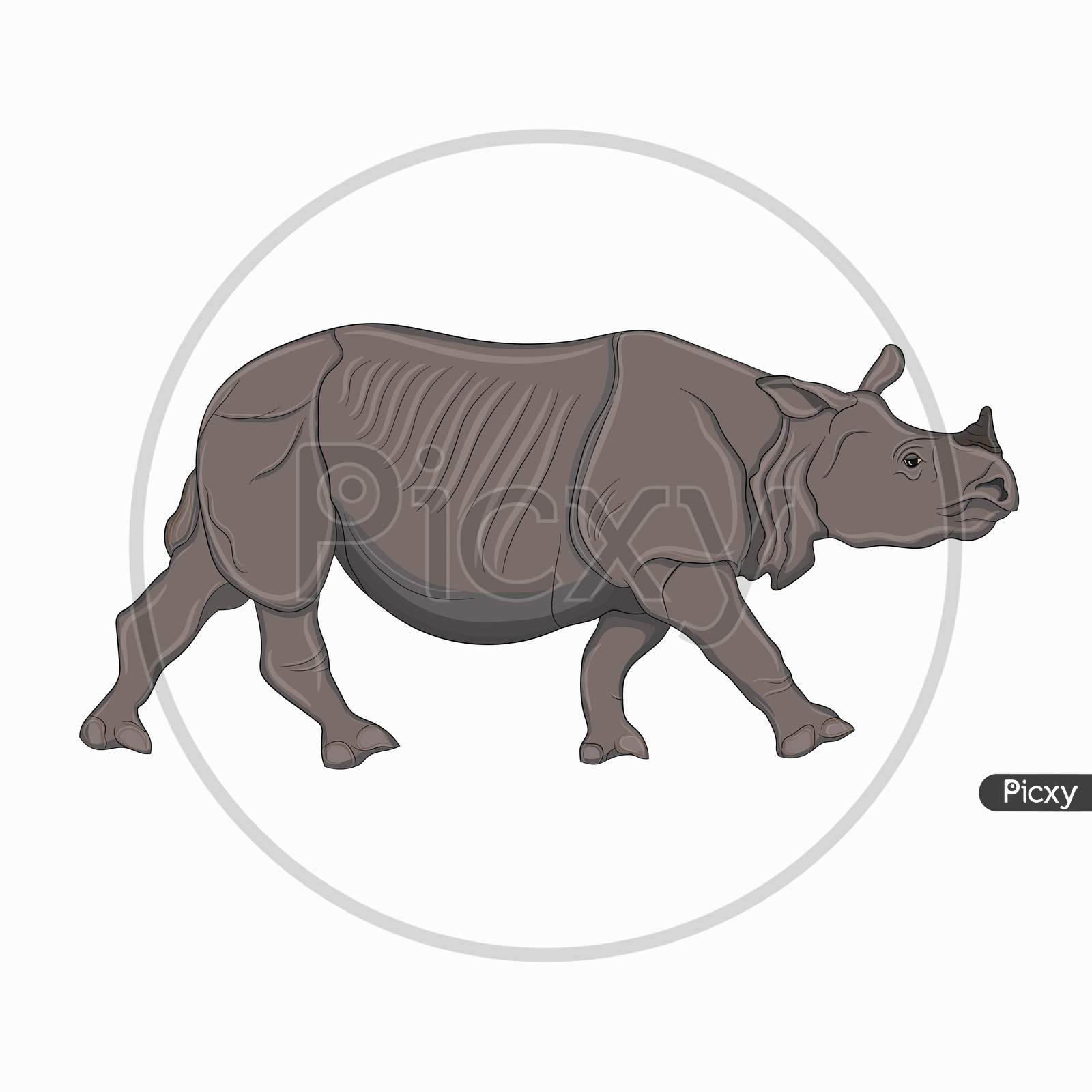The image, set against an off-white background, features a simple, cartoony illustration of a rhinoceros in a walking motion facing to the right, showcasing its detailed, textured gray-brown body. The rhinoceros, complete with a small, darker bump-like horn atop its snout, is depicted in profile, highlighting the thick skin typical of the animal through visible linework. Encircling the majority of the rhino, except for its nose and back leg, is an opaque gray circle with a white outline, which partially intersects with its body. Prominently displayed across the rhino is a gray watermark with a white outline, reading "PICXY". Additionally, the word "PICXY" appears both on the left and right sides of the circle in white font.